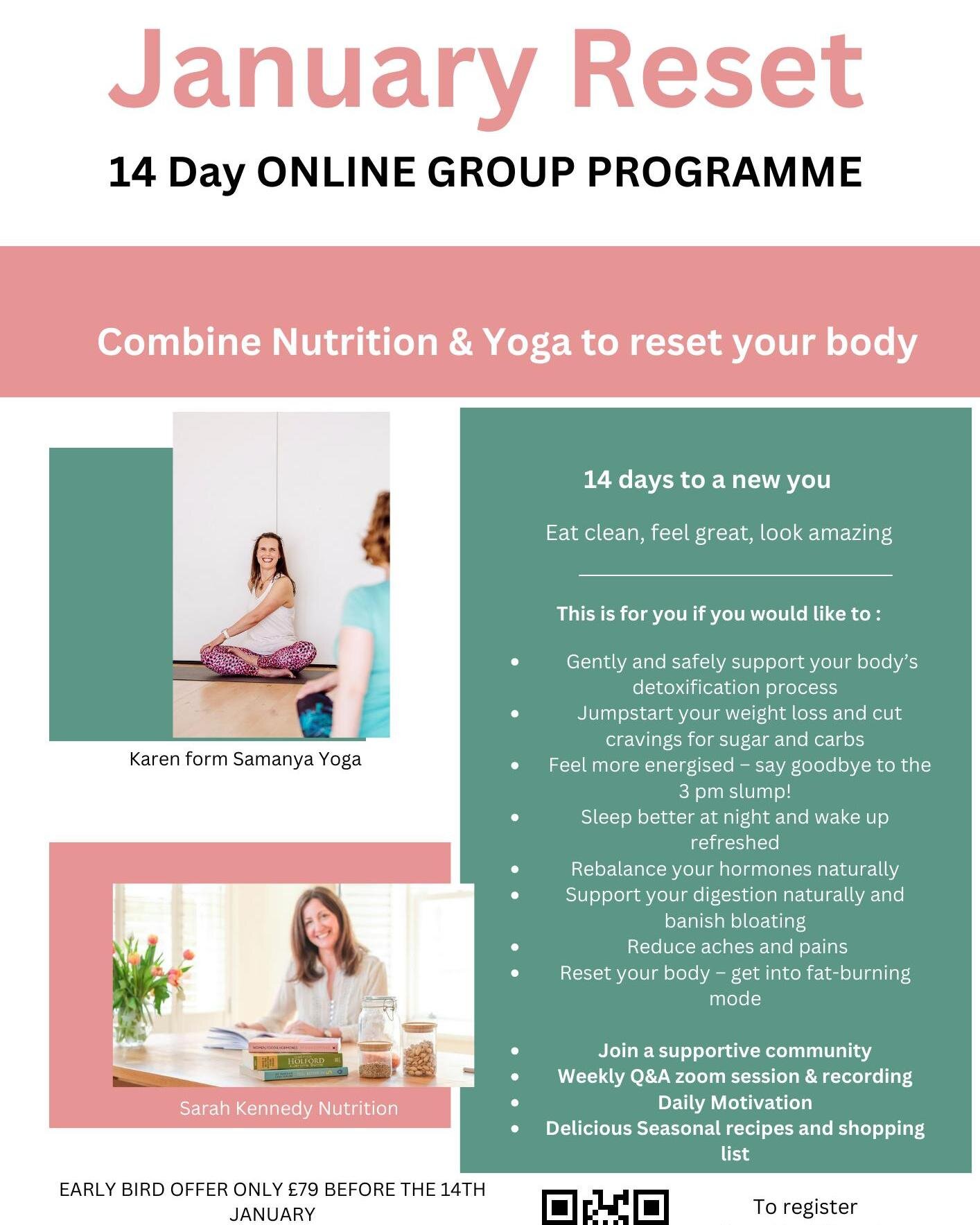**Caption:**

"Join the January Reset: A 14-Day Online Group Program (British English spelling) to rejuvenate your body and mind. This comprehensive program combines the best of nutrition and yoga, with expert guidance from our seasoned instructors. 

Featured on the flyer are two authentic images of our dedicated teachers: on the left, Karen, a certified instructor from Samanya Yoga, ready to guide you through restorative yoga sessions, and on the right, Sarah Kennedy, a specialist in nutrition to help you adopt clean eating habits. 

Embark on this journey to a new you with daily yoga classes and personalized nutrition plans designed to detoxify your body, enhance fat-burning, and boost your overall well-being. 

Sign up now to experience the transformational benefits of combining mindful movement and nutrition."